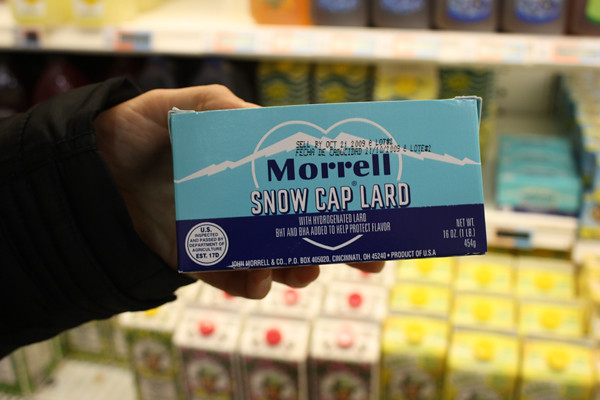The image is an indoor color photograph showing a close-up of a person's left hand, which is wearing a long-sleeved black jacket and holding a rectangular box of Morrell Snow Cap Lard. The box, which is reminiscent of boxed butter, features a distinctive design with the upper two-thirds in light blue showcasing an outline of a snow-capped mountain and a heart, and the lower third in a darker navy blue. Prominently written in dark blue in the center of the box is the brand name "Morrell" followed by "Snow Cap Lard" in white letters. Further details on the box include the text "Morrell Snow Cap Lard with hydrogenated lard, BHT, and BHA added to help protect flavor," a "Sell by October 21, 2009" date, and a U.S. inspected stamp in a circle. The background reveals part of a grocery store aisle, with various products blurred out, and additional boxes of similar lard. The shopper's hand centers the product in the image, emphasizing the detailed packaging.